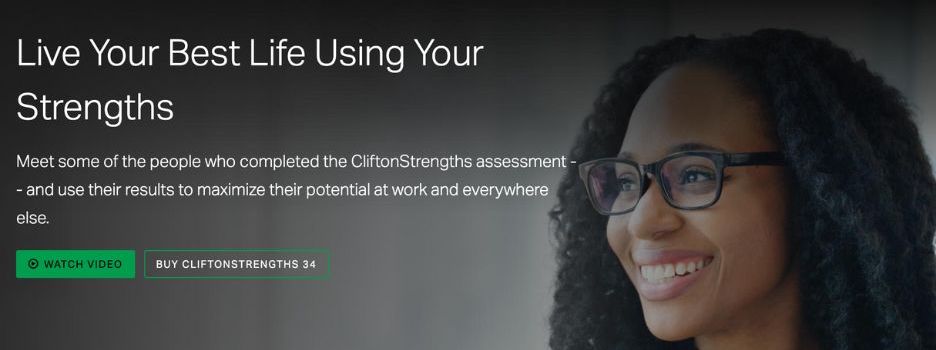The image depicts a section of a website page, specifically the middle left portion. At the top left, a large, white-font heading reads, "Live Your Best Life Using Your Strengths." Below this heading, the accompanying text states, "Meet some of the people who completed the CliftonStrengths Assessment and use their results to maximize their potential at work and everywhere else." The term "CliftonStrengths" is presented as one unified word.

Beneath the text, there are two distinctive rectangular areas. The first, on the left, contains the phrase "Watch Video" alongside a circular play button. To the right of this, another elongated rectangle displays the text "Buy CliftonStrengths" and includes the number 34. The background color of these elements matches the overall image, which transitions from a darker gray on the left to a lighter shade.

Dominating the right side of the image, there is a photograph of an African-American woman. She is gazing to her right, sporting black glasses, and has shoulder-length, curly hair. The image captures her from the neck up, showcasing her smile, with her cheeks raised and her eyes exuding vibrancy and joy.